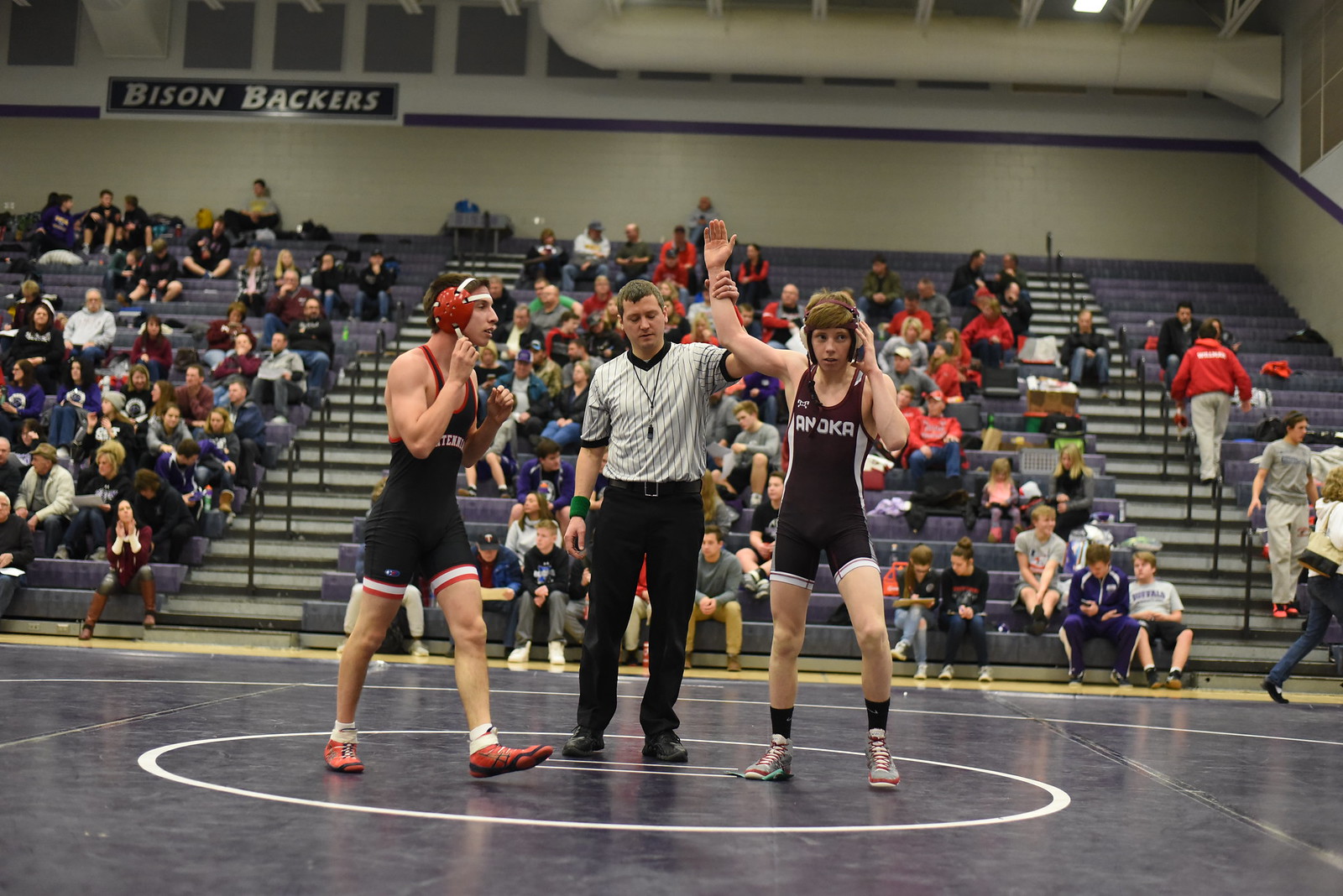This detailed photograph captures an indoor wrestling match featuring two young male wrestlers positioned at the center of the image, alongside a referee who is raising the arm of the boy on the right, indicating his victory. The wrestlers are on a hard, shiny surface that appears painted, possibly marking a wrestling mat or court. The background features bleachers that are partially filled with spectators. Above the bleachers, a sign reads "Bison Backers." The venue’s interior is characterized by beige walls with blue trim, transitioning to white and gray near the ceiling, where a large ductwork tube is visible. The scene is set amidst an active wrestling match, likely taking place at night in what appears to be a gymnasium. The color palette of the image includes black, white, red, tan, maroon, orange, blue, green, and gray.